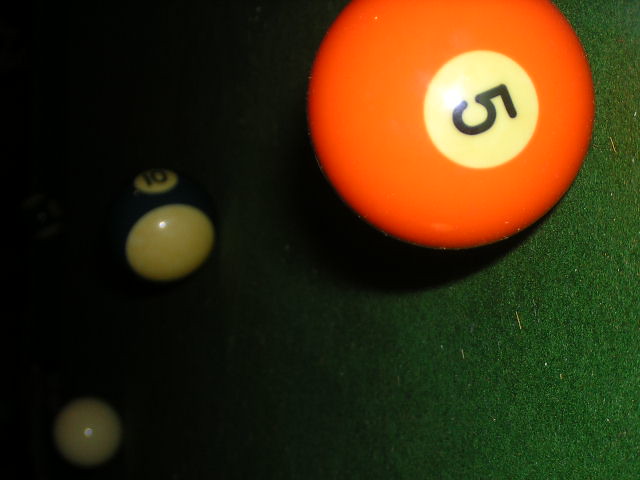In this artfully composed photograph that exudes a nostalgic 70s vibe, three pool balls are positioned on a green felt pool table. The primary focus is on a bright orange billiard ball marked with the number 5, situated in the top right corner, slightly tilted to the right. The pool table's green felt appears to have a light shade, likely enhanced by the flash. In the back left corner, a partially visible striped number 10 ball, with a white background, sits in a darker area of the table, adding a sense of depth. Behind this, nestled in the darker section of the table, a white ball shimmers faintly, its precise details obscured by the shadow. The overall scene, viewed as though rotated counterclockwise, creates an intriguing and detailed study of the colorful billiard balls and their vintage setting.